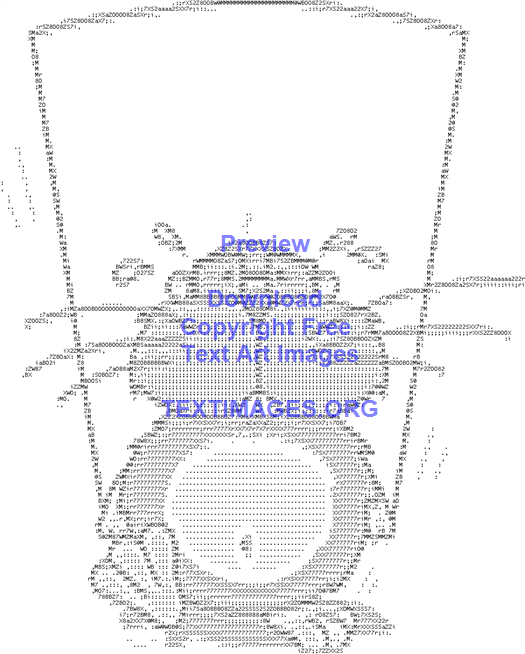The image is a detailed ASCII art illustration featuring a small rodent-like creature, potentially a hamster, mouse, or beaver. The creature has long whiskers—three on each side of its face—and appears to be sweating with beads of perspiration on its head, giving it a nervous or worried expression. Its rounded stomach and light-colored three-toed feet add to its distinct, cartoony style. The rodent is depicted walking forward while holding a large, arced container with narrowing sides, possibly a glass or basket, in its hands. This intricate artwork is created using text, numbers, symbols, and characters meticulously arranged to form the image. Superimposed over this image in blue font are the words: "Preview, download, copyright-free text art images," and then "textimages.org."